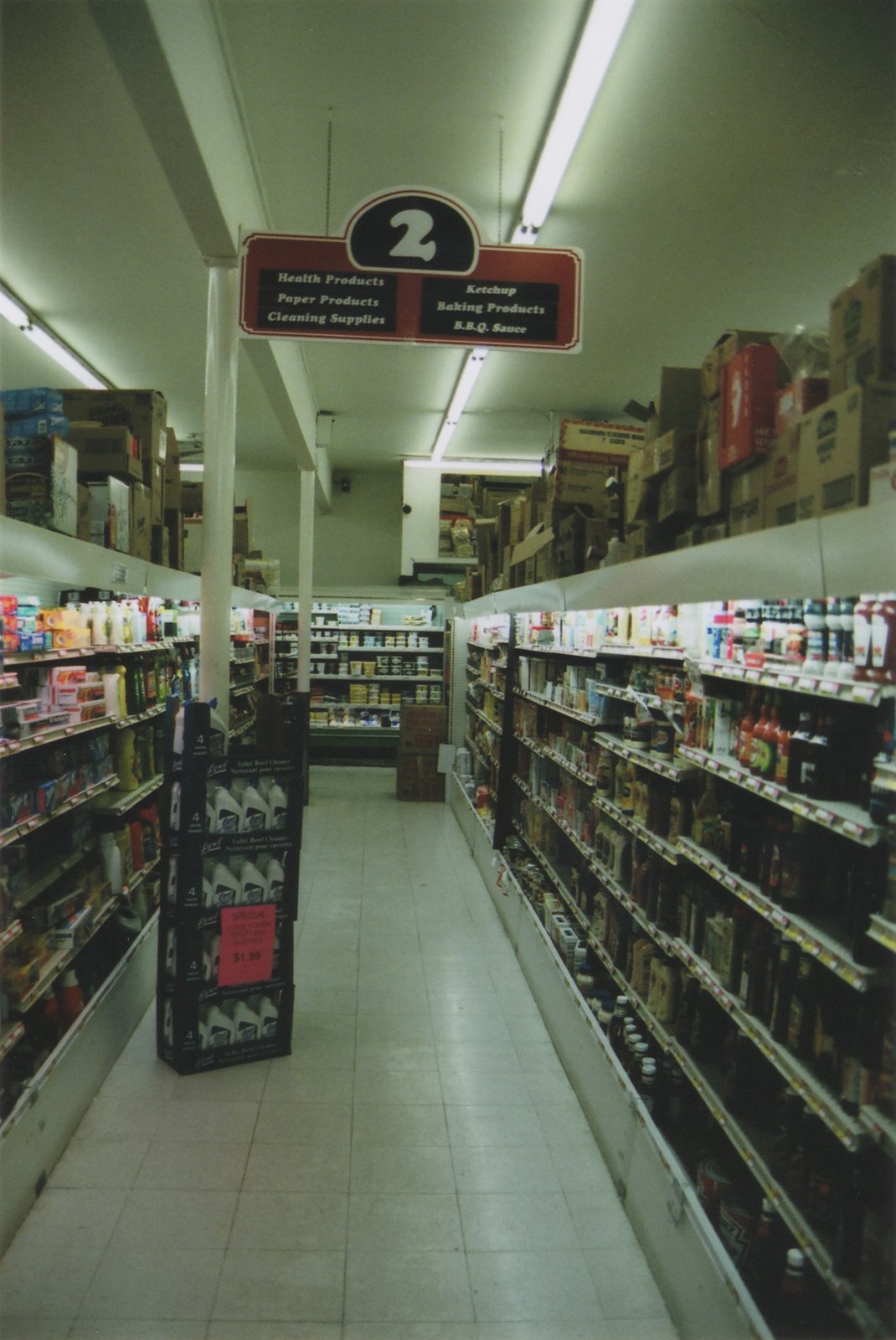This grainy photograph, likely from an earlier era, captures the interior of a store with remarkable detail. The image foregrounds two prominent aisles stocked with an array of diverse products, while another aisle is discernible in the background. A sign, suspended near the ceiling, features a large white number "2" against a black background, accented with subtle red trim. Below this, the main section of the sign showcases a red backdrop interspersed with black rectangles bearing white font. Fluorescent lights illuminate the scene, reflecting off the white tiled floors that stretch across the store. The aisles burst with color, featuring an assortment of products, including multiple food jars sporting hues of blue, red, yellow, gold, black, and green. On the side of the image, a plastic display case houses white and blue bottles, topped with a red sign, contributing to the photograph's rich visual narrative.